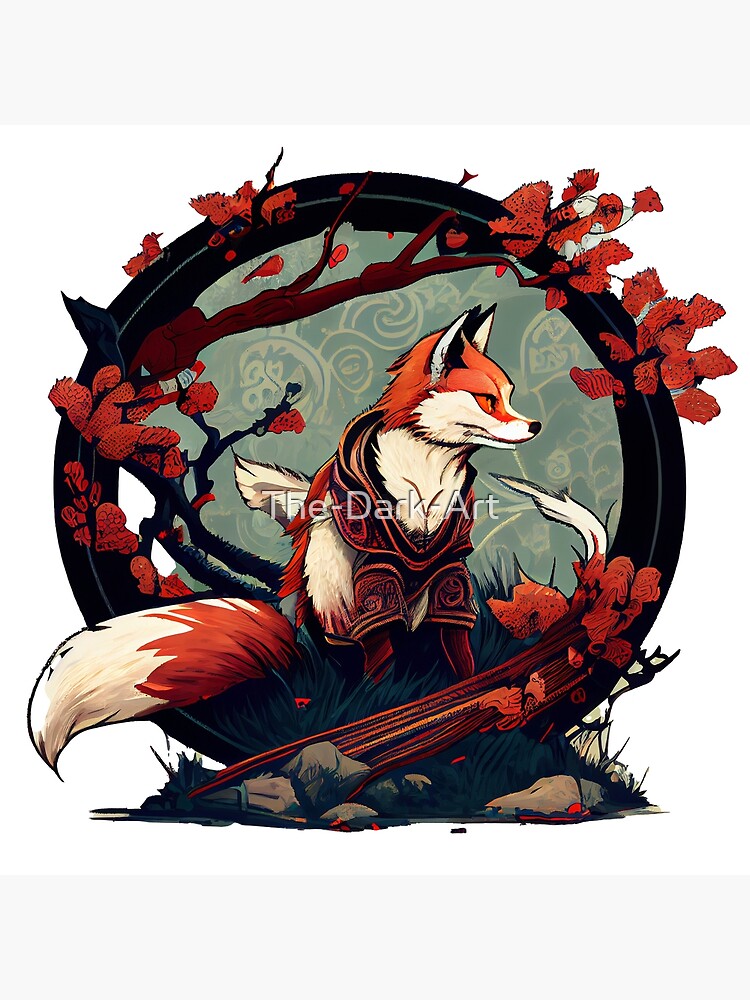This detailed image depicts a digital artwork centered around a stylized red and white fox. The fox is seated inside a thick black circular wreath adorned with orangish-red leaves and tree branches that stretch across the top. The fox, facing to the right with its bushy tail extending to the left, showcases pointy ears trimmed in black, a black nose, and a mix of red and white fur. Adding to its artistic charm, the fox appears to be wearing a harness or shirt with black trim and swirly patterns around its neck and front legs. This central motif rests atop a mound of dark green and black grasses interspersed with small gray rocks. The background within the wreath features a pale bluish-green area filled with artistic swirls and light gold filigree designs. Atop the image, a subtle watermark reads "the dark art," highlighting the digital nature of this captivating artwork.